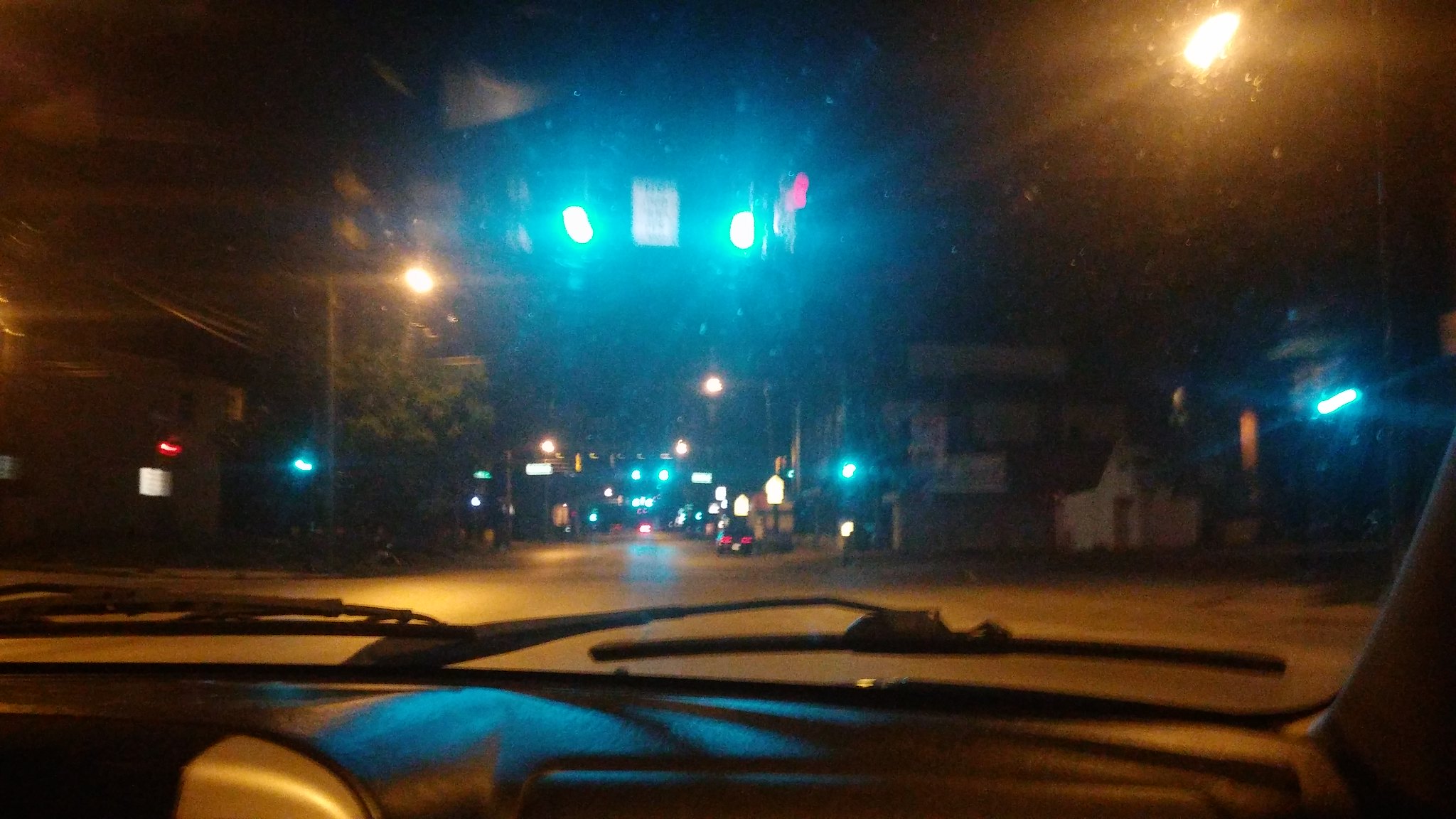This nighttime photograph, taken from the passenger side inside a car, captures an urban street scene through the windshield. The dashboard and the glove box outline are visible in the foreground, along with two flattened black windshield wipers. The windshield itself has noticeable spots. Ahead, a series of green traffic lights extend down the street, creating a sense of depth, with a multitude of intersections visible. The closest intersection features a blurry red arrow and a white traffic sign, potentially indicating restrictions like "no turn on red." 

The image reveals faint, shadowed buildings against the dark sky, illuminated intermittently by yellow and orange streetlights on either side of the street. To the upper right, a luminescent yellow streetlight shines brightly, while to the left, small red and blue lights add to the city’s nightscape. The blur in some areas suggests either movement or the quality of the camera, adding to the lively yet hazy ambiance of the urban night.